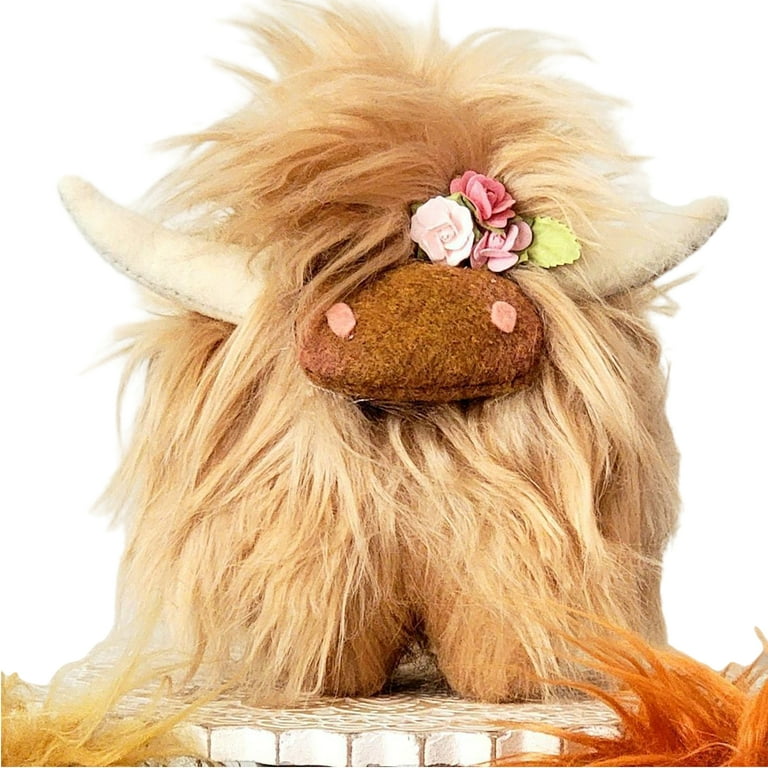The image depicts a stuffed animal that resembles a Highland cow with long, yellowish-blonde fur that cascades over its eyes and body. The plushie sits atop a tiled plate with gear-like teeth along its edge and ornate printing on its surface. This Highland cow features two prominent horns extending from either side of its head and sports a small bundle of roses on the top of its nose. The roses vary in shades from white and pale pink to deep pink, accompanied by a yellow leaf. The animal’s nose is marked by two small buttons, adding to its charming appearance. In the background, two other stuffed animals slightly encroach into the frame, their fur visible on the lower left and right edges. The entire scene is set against a plain white backdrop, devoid of any text or additional elements.